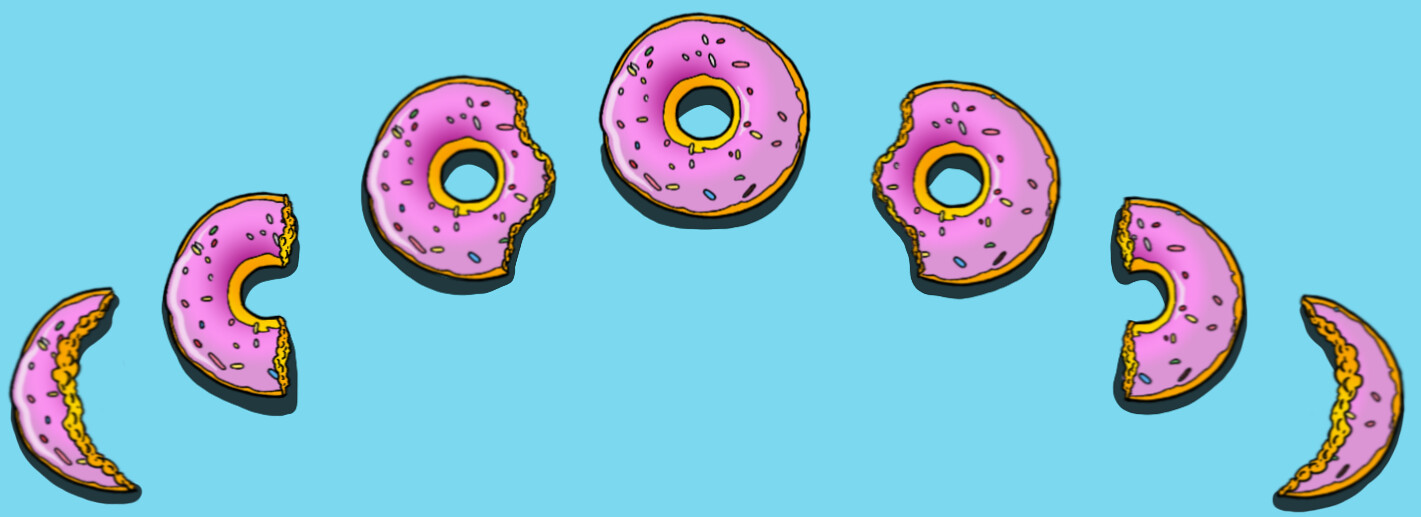This illustration features an arrangement of pink frosted ring biscuits with colorful sprinkles, set against a uniform sky blue background. The composition follows a symmetrical pattern, resembling the phases of the moon, with the biscuits becoming progressively more complete toward the center and then reversing back to a crescent shape. At the center top of the image, a fully intact pink frosted biscuit with a hole in the middle is depicted. On either side, extending outward, the biscuits show progressively more bites taken out of them. The first set of biscuits next to the central one have a bite on opposite sides—right side of the left biscuit and left side of the right biscuit. As the pattern continues, the biscuits become half-moon shapes, with the left biscuit missing its right half and the right biscuit missing its left half. At the far edges of the image, only crescents of the biscuits remain, with substantial portions eaten away. The inside of each biscuit is yellow, adding a contrast to the pink icing and colorful sprinkles on top. The depiction creates a visual gradient from partially eaten to whole and back to partially eaten, capturing the progression of consumption in a visually appealing manner.